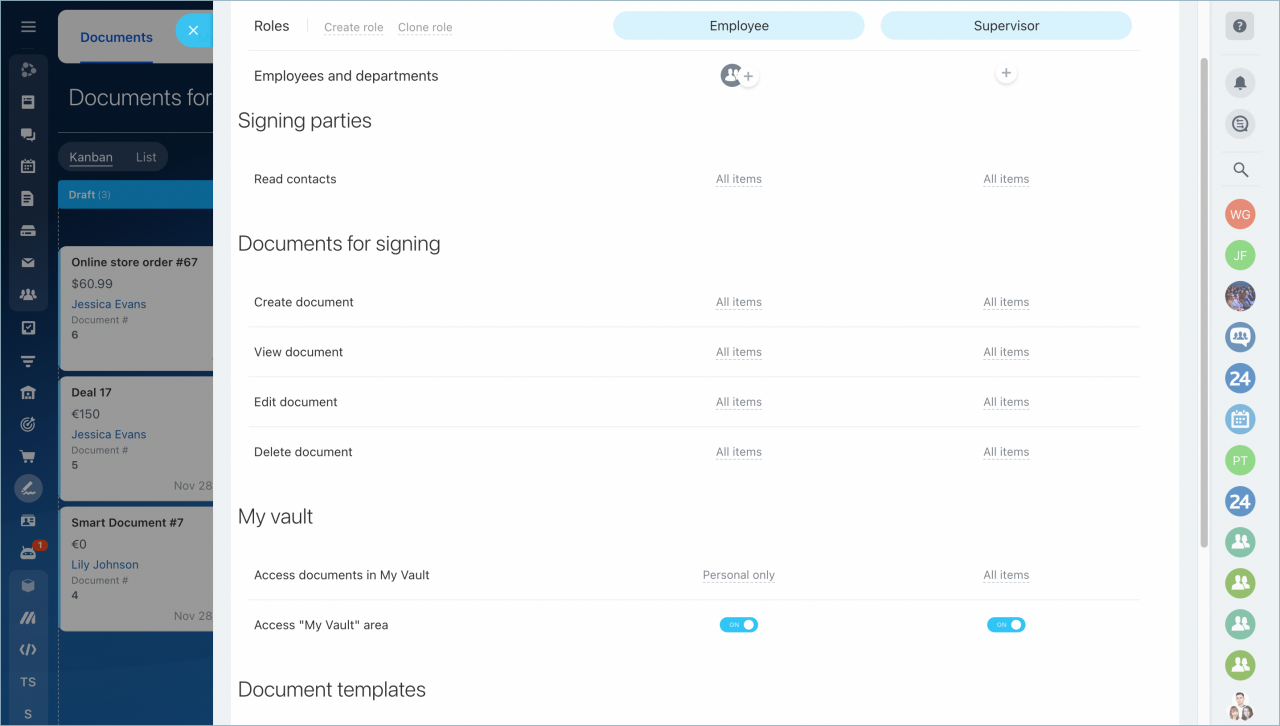The image appears to be a screenshot of a business-oriented software interface. On the left side of the screen, the background is a dark blue color, displaying several entries: "Documents," "Kanban List," "Draft," and various records pertaining to orders and deals such as "Online Store Order 67" priced at $60.99, associated with Jessica Evans; "Deal 17" valued at 150 Euros, also linked to Jessica Evans; "Smart Document No. 7" costing 0 Euros, associated with Lily Johnson; and "Document No. 4."

The central focus of the image is contained within a white background at the top featuring a navigation bar. The header "Roles" is in black, accompanied by light gray options "Create Role" and "Clone Role," which are unselected. There are light blue ovals labeled "Employee" and "Supervisor."

Below this, a section titled "Employees and Departments" is present, along with a gray circle icon featuring a people symbol and a plus sign. The "Supervisor" section similarly features a circle with a plus sign. The subsequent categories include "Signing Parties" and "Read Contracts." Both columns under "Employee" and "Supervisor" have entries labeled "All Items."

Further down, the section "Documents for Signing" lists the actions "Create Document," "View Document," "Edit Document," and "Delete Document" vertically. Adjacent to each action, under both "Employee" and "Supervisor" columns, it reads "All Items."

To the left, "My Vault" is indicated with the note "Access Documents in My Vault." In the "Employee" section, it specifies "Personal Only," while in the "Supervisor" section, it mentions "All Items." The term "My Vault" is placed within quotation marks, with a light blue oval featuring a white dot to the right in both columns.

The final section labeled "Document Templates" is empty, with no additional information provided beneath it.